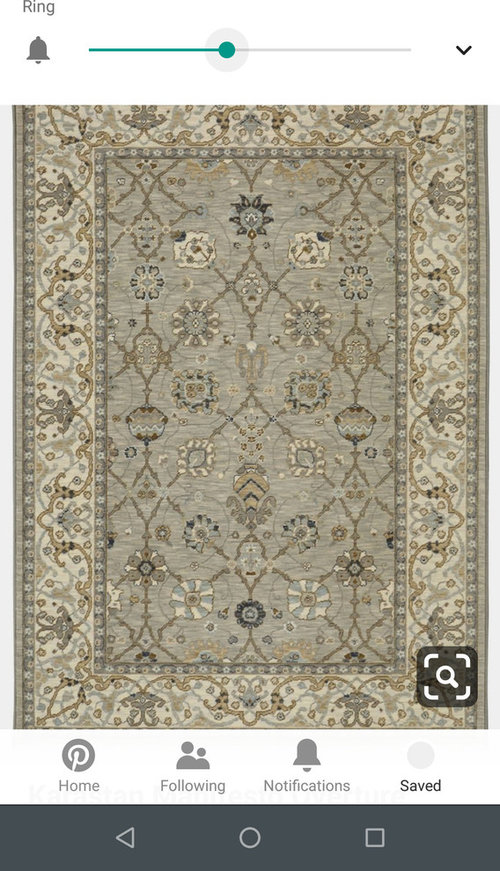The image is a detailed close-up view of a multi-colored rug displayed on a phone screen. The rug features a diverse palette of tones, including various shades of beige, subtle grays, rich browns, hints of burnt yellow, touches of white, and darker accents like black and dark gray.

At the upper left corner of the screen, there's a small gray bell icon with the word "ring" positioned above it. Below this, a horizontal line spans from the left to right, with the left segment being green and featuring a central green dot. An arrow points downward nearby.

The majority of the image is occupied by the intricate patterns of the rug. Additional interactive screen elements are present: a magnifying glass icon for zooming in on the rug image, and buttons labeled "Pinterest," "Home," "Following" (accompanied by an icon of two people), "Notifications" (next to a bell icon), and "Saved" (adjacent to a circle icon).

At the very bottom of the screen, a black rectangular navigation bar is visible, featuring a triangle on the left, a circle in the middle, and a square on the right.